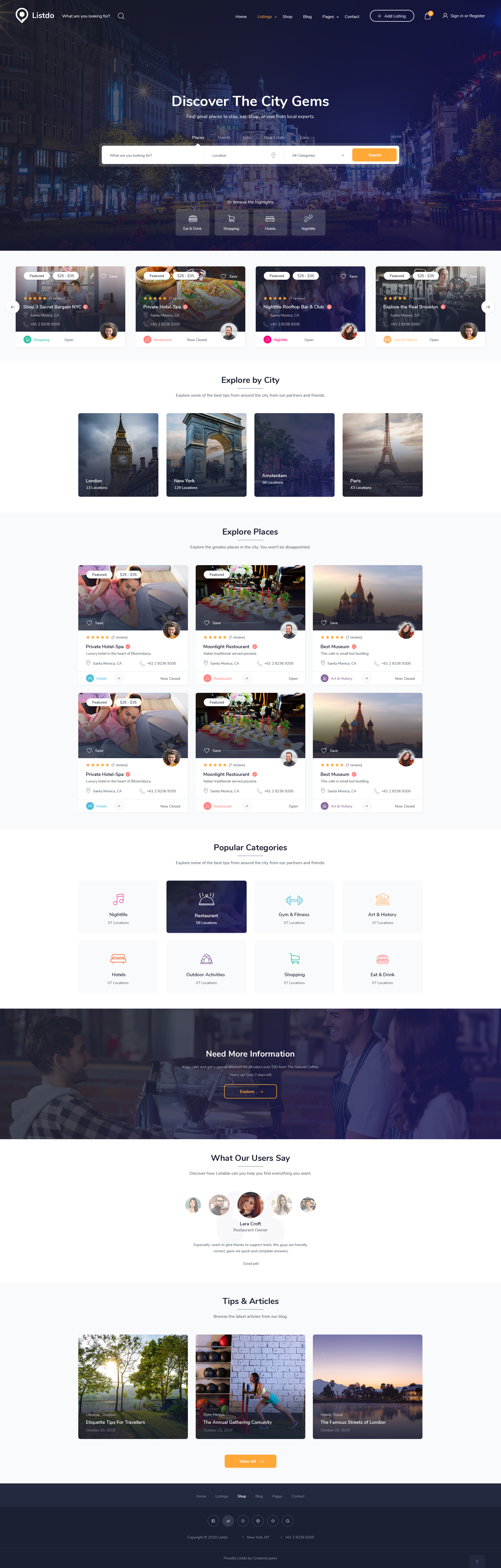This screenshot captures a webpage from the website ListDo, prominently displayed in the upper left corner. Despite the small size of the image, the main elements are discernible. 

In the upper right corner, there are options to sign in or register in white text. The top portion of the page features a banner with a nighttime city scene encompassing buildings on either side and what appears to be a road in the center. Central to this scene, in bold white text, is the phrase: "Discover the City Gems. Find great places to stay, eat, shop, or visit from local experts."

Below this banner, a prominent white search bar invites users to enter a location and specify what they are looking for, with the search command highlighted in a yellow rectangle. Directly beneath this search bar is a section titled "Browse the Highlights," which includes four gray boxes. The first box on the left, with an image that appears to be a hamburger or hot dog, is labeled "Eat and Drink." Next to it is a box with a shopping cart icon labeled "Shopping," followed by "Hotels," and lastly what is likely "Highlights."

Further down, against a white background, are images of various places to eat. Text for these images includes "Shop Three Secret Bargains NYC," "Private Hotel Spa," "Nightlife Rooftop Bar and Club," and "Explore the Real Brooklyn."

At the bottom of the image, there is another section featuring four color photographs under the header "Explore the City." Each photograph represents a different city scene: London, New York, Amsterdam, and Paris, from left to right.